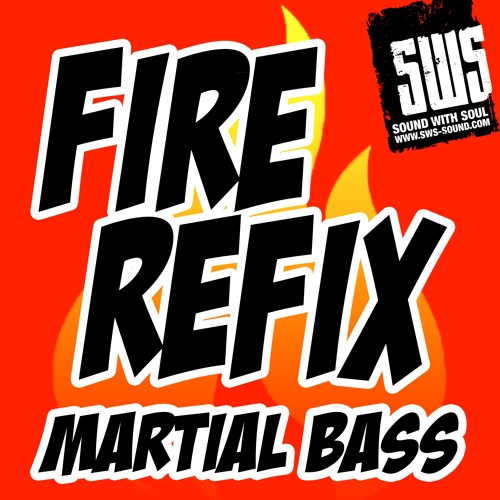The promotional image showcases a vivid, solid bright red background with striking, orange flame graphics radiating from the center. Dominating the center is bold black text with a white border that reads "FIRE REFIX" in a large, hand-designed font, with "MARSHALL BASS" written in smaller, all-caps lettering below it. In the top right corner, there's a slightly angled, black square logo with white text that boldly states "SWS," followed by "Sound with Soul" and the website "www.sws-sound.com." The captivating combination of typography and graphic design effectively creates a dynamic and intense visual, perfect for promoting the band or music event.